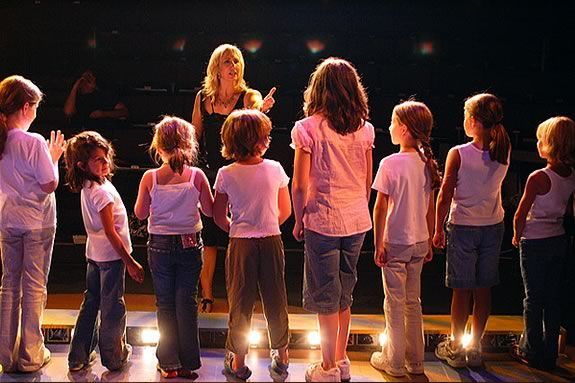The photograph captures a rehearsal scene on a stage, featuring a group of nine young girls viewed from behind, standing in a horizontal line. The girls, who primarily wear white tops and blue jeans with some variations in the bottoms, appear to be receiving instructions from a middle-aged Caucasian woman positioned at the front, facing them. The instructor, dressed in a black knee-length dress and with blonde hair, has her left hand raised with her pointer finger extended, as if giving detailed directions. Her expression seems focused and perhaps a bit frustrated. The stage is brightly lit, with five lights along the floor illuminating the girls and additional overhead lighting focusing on the teacher. In the background, the dimly lit auditorium reveals the outlines of empty chairs and a couple of indistinct figures, emphasizing that this is likely a practice session for an upcoming performance. The overall setting suggests a structured, instructive environment, likely related to theater or choir practice.